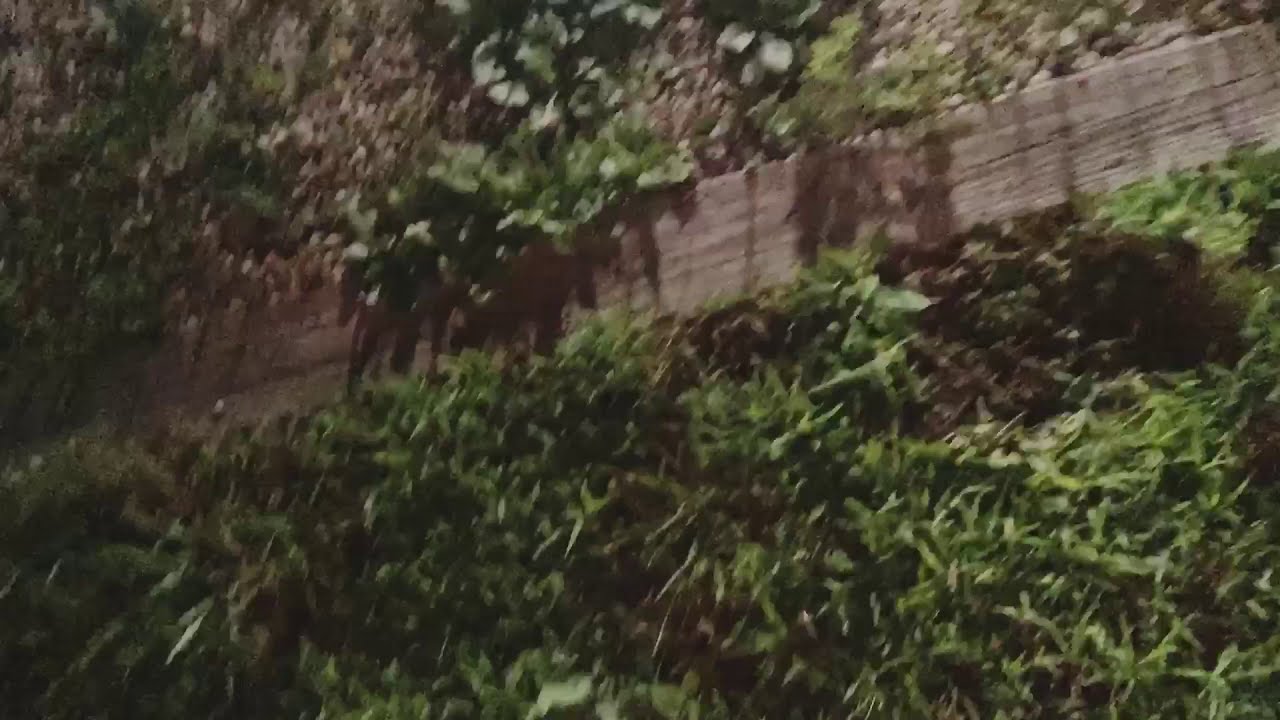The image depicts a blurry, nighttime scene, likely taken from a video, showing a patch of natural grasses and various plants. The camera angle suggests it is being held by someone standing, looking down from a higher elevation. Illuminated primarily by a nearby lamp post or street light, the scene is characterized by muted earth tones—greens, browns, blacks, and grays—accentuating its dimly lit environment.

Central to the composition is a single wooden plank running diagonally from the bottom left to the top right of the image. This divider appears to separate an area of patchy grass and dried shrubs from a section of loose stones. The ground around the plank seems somewhat uneven, with possible depressions indicative of a marshy texture or areas where plants have been uprooted.

This likely outdoor setting could be part of a garden, a backyard, or a walkway beside a house, where the wooden board serves to prevent walking directly on the potentially muddy ground. The presence of small weeds among the stones suggests a natural, unmaintained area, possibly designed to keep vegetation from encroaching on the pathway.